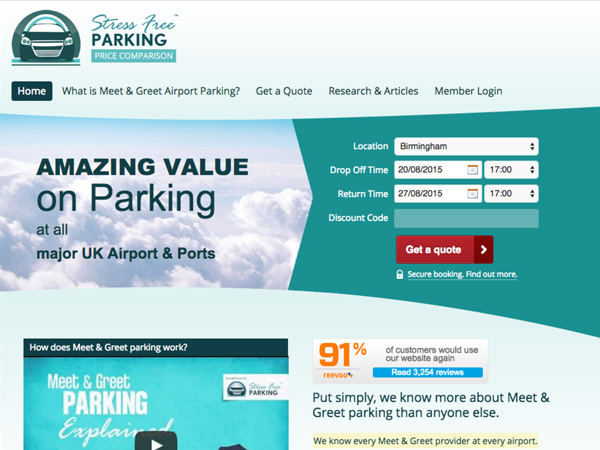This image is a screenshot of the home page from a stress-free parking price comparison website. The focal point of the page is a section where users can get a quote for parking in various locations across the UK, specifying drop-off and return times, and applying discount codes for cheaper parking options at all major UK airports and ports. An embedded video on the page explains the functionality of meet and greet parking services. Navigation headers at the top of the page direct users to different sections, including a detailed description of meet and greet airport parking, a page for obtaining quotes, a research and articles section, and a member login area. The page is designed in color but features a subdued palette. There are no people depicted in the screenshot. Additionally, there is a link available for users to read reviews from past customers, enhancing the credibility and user experience of the website.